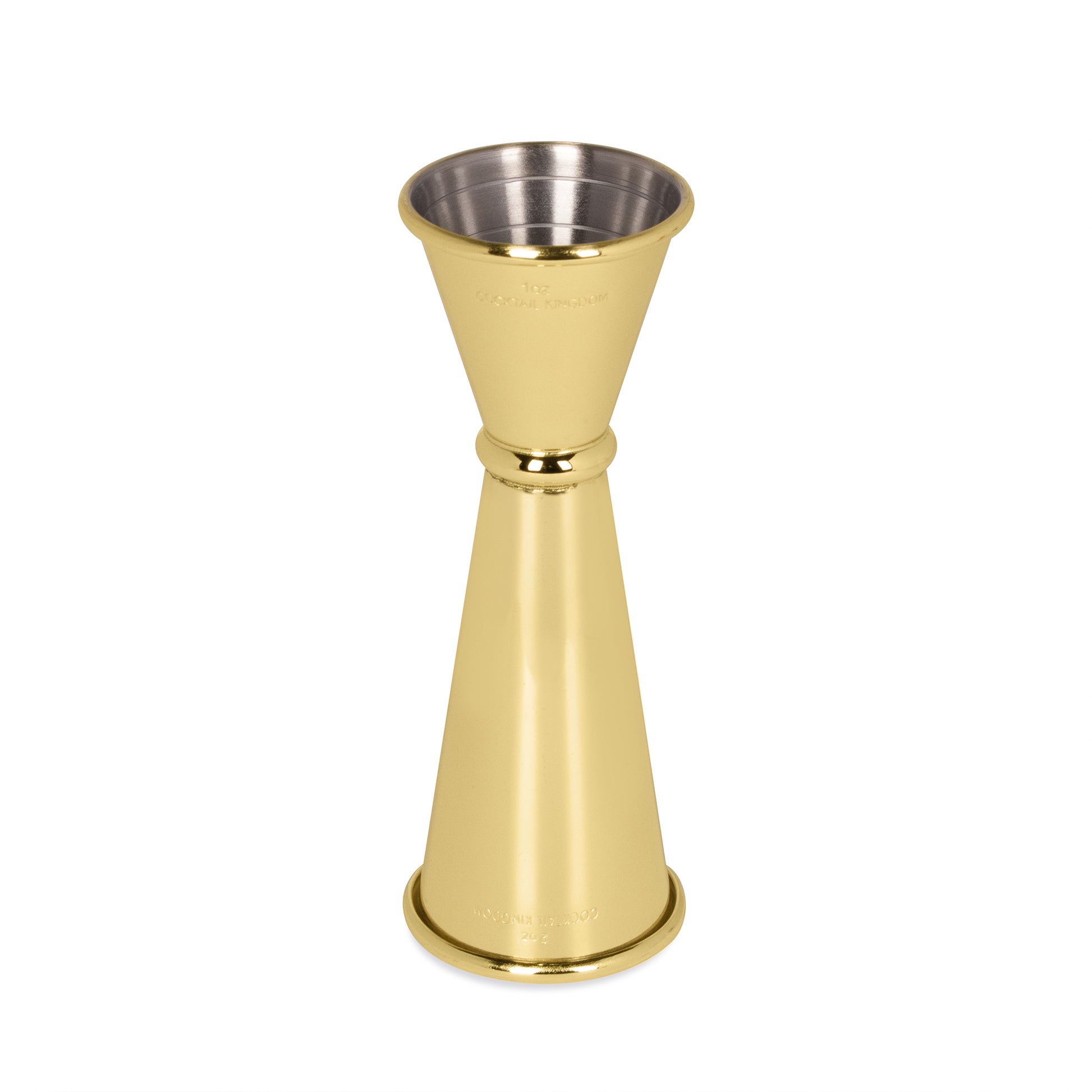In this image, there is a double-sided shot measuring tool that appears to be used by bartenders for mixing drinks. The exterior is a glossy, metallic gold or brass, while the interior is a contrasting silver, possibly made of stainless steel or aluminum. The device has two ends of different sizes; one end is likely for measuring one ounce and the other for two ounces, as indicated by faint markings inside. The tool stands out prominently against a completely white background, emphasizing its polished, shiny appearance. The absence of any additional objects or colors in the background highlights the tool's functionality and sleek design.